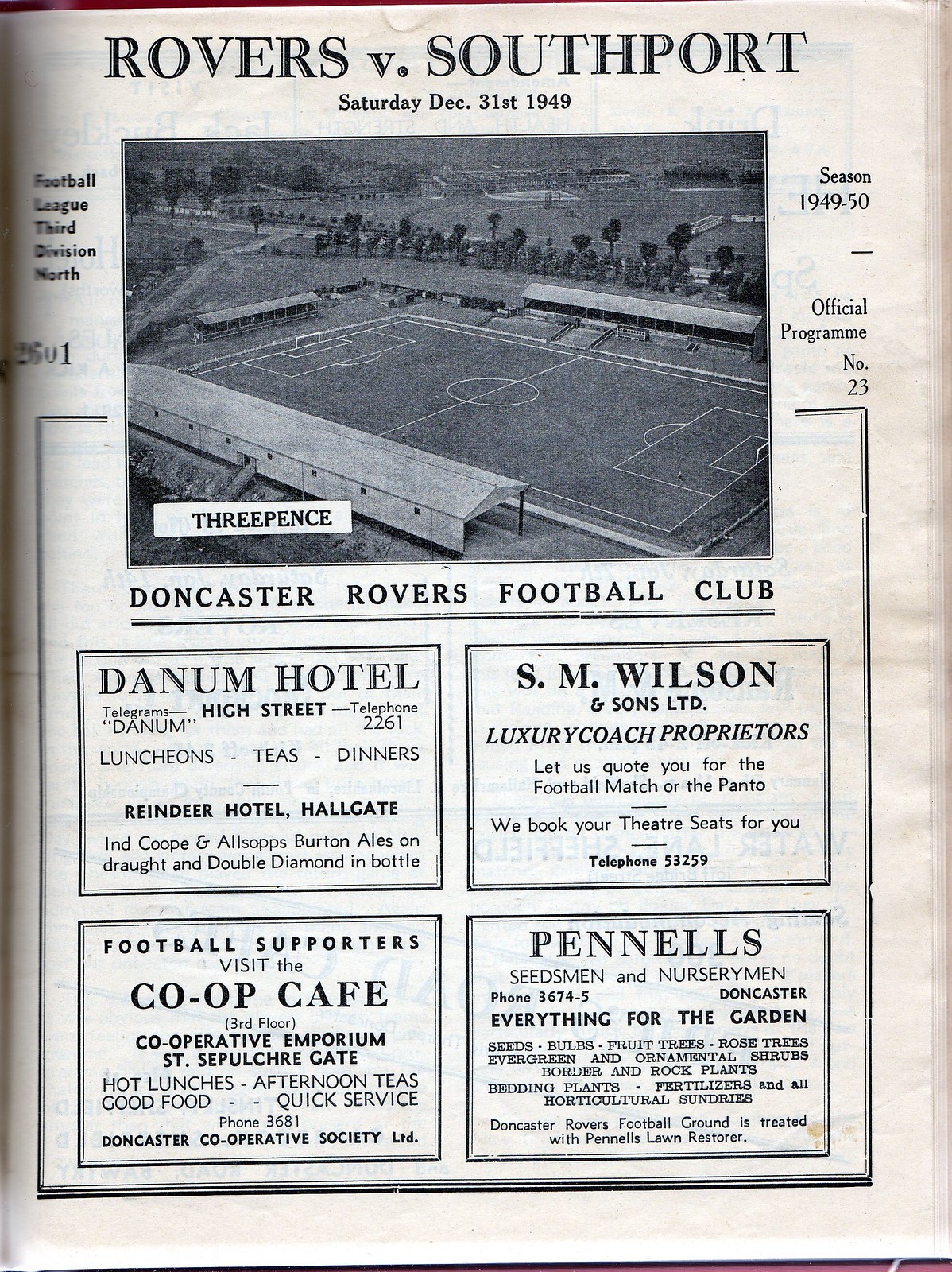This black-and-white scanned image of a vintage football program from the 1949-50 season features a match between Rovers and Southport, dated Saturday, December 31st, 1949. The program is for the Football League, 3rd Division North and is numbered 23. At the top of the image are the match details, followed by a picture of the soccer field. The bottom of the picture is labeled "3 pence." On the left side of the image, it indicates "Football League, 3rd Division North," while the right side reads "1949-50 season, official program, number 23." Below the picture, the central text declares, "Doncaster Rovers Football Club." Surrounding this central text are four advertisement squares: 

- The top left square advertises Danum Hotel, High Street, with contact information and details about their Luncheons, Teas, Dinners, Reindeer Hotel, Hallgate, and Alsop’s Burton Ales.
- The top right square highlights S.M. Wilson and Sons, Ltd., offering luxury coach services for football matches or theatre visits, including booking services.
- The bottom left square promotes Football Supporters visiting the Co-op Cafe at the 3rd Floor, Co-operative Emporium Street, Sepulcher Gate, known for its quick service and good food.
- The bottom right square features Pennells, Seedsmen, and Nurserymen in Doncaster, detailing their extensive range of gardening supplies and noting that Doncaster Rovers Football Ground uses Pennells Lawn Restorer.